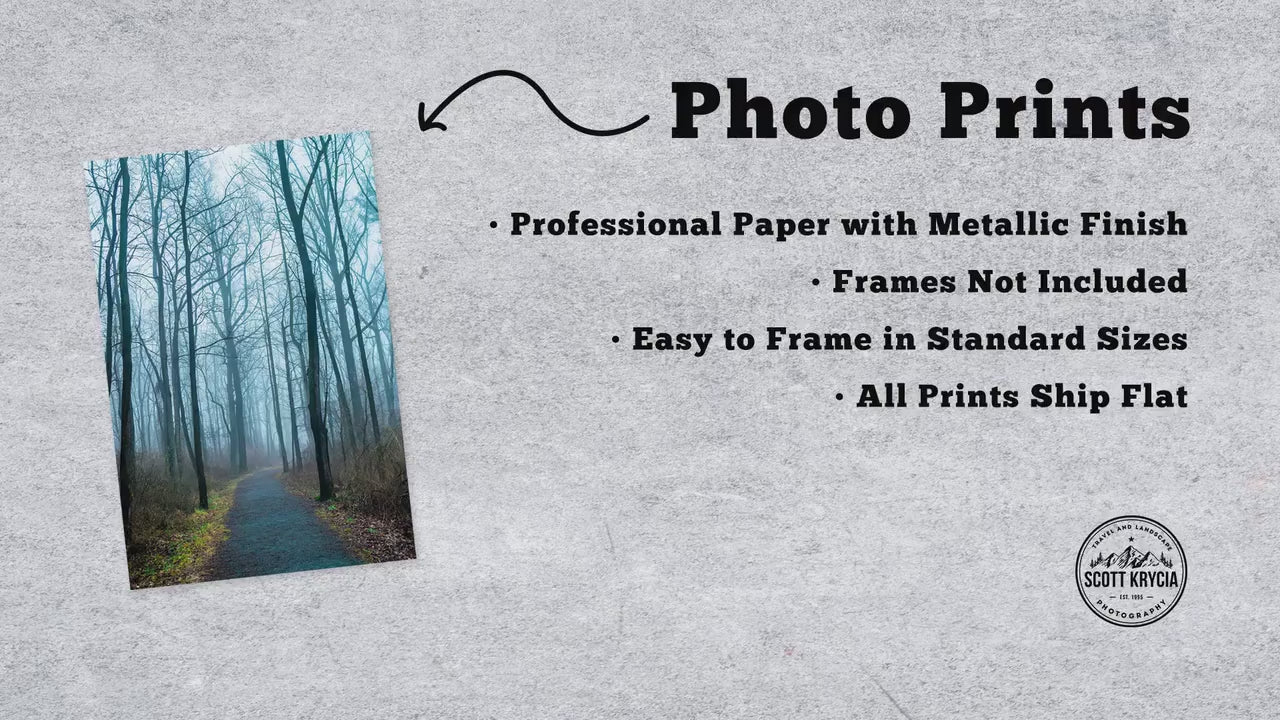The rectangular advertisement features a mottled, textured gray background that resembles gray paper or a computer-generated marble effect. Dominating the left side is a tall, rectangular photograph showcasing an asphalt walkway cutting through a leafless, foggy forest, where the black and gray trunks of skinny trees stretch upwards. Some fallen yellow and orange leaves are scattered beneath the trees, reinforcing an autumnal atmosphere. To the right of the photograph, an arrow points towards it, labeled "Photo Prints" in large black text. Below this, several bullet points in an easy-to-read black font detail the product features: "Professional paper with metallic finish," "Frames not included," "Easy to frame in standard sizes," and "All prints ship flat." In the bottom right corner, a circular logo displays a simple drawing of mountains above the name "Scott Krycia Photography," with additional smaller text and "Est. 1990" that are too small to read clearly.